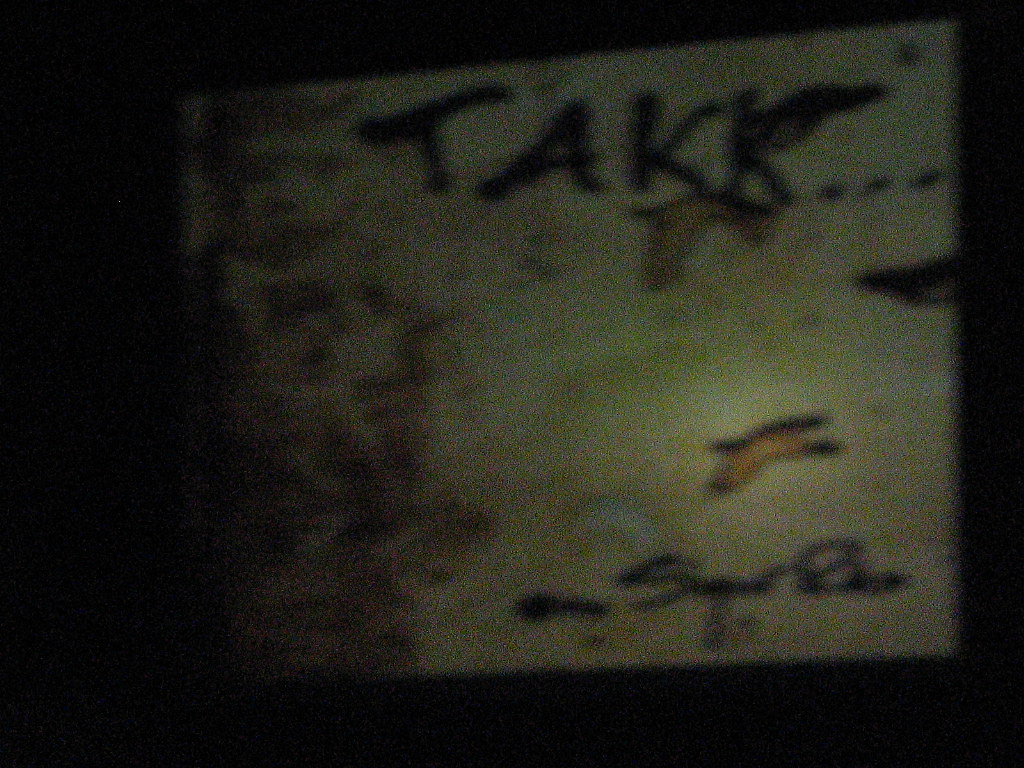The photograph is a rectangular image presented in a landscape orientation, with a solid black background that starkly contrasts the featured object. Central to the composition is a slightly tilted, smaller rectangular object, positioned upwards and to the right relative to the frame. This object is an off-white color, lending a vintage or worn appearance. Prominently displayed at the top of this object are the bold, black letters "T-A-K-K," followed by an ellipsis, hinting at an unfinished thought or continuation. Near the bottom of the object, there is a word that remains indistinct and difficult to decipher. Adding to its weathered aesthetic, the object is marked with several dark gray and brown spots of varying sizes, suggesting age, use, or exposure to elements. The overall composition is minimalistic yet textured, evoking curiosity about the object's history and purpose.